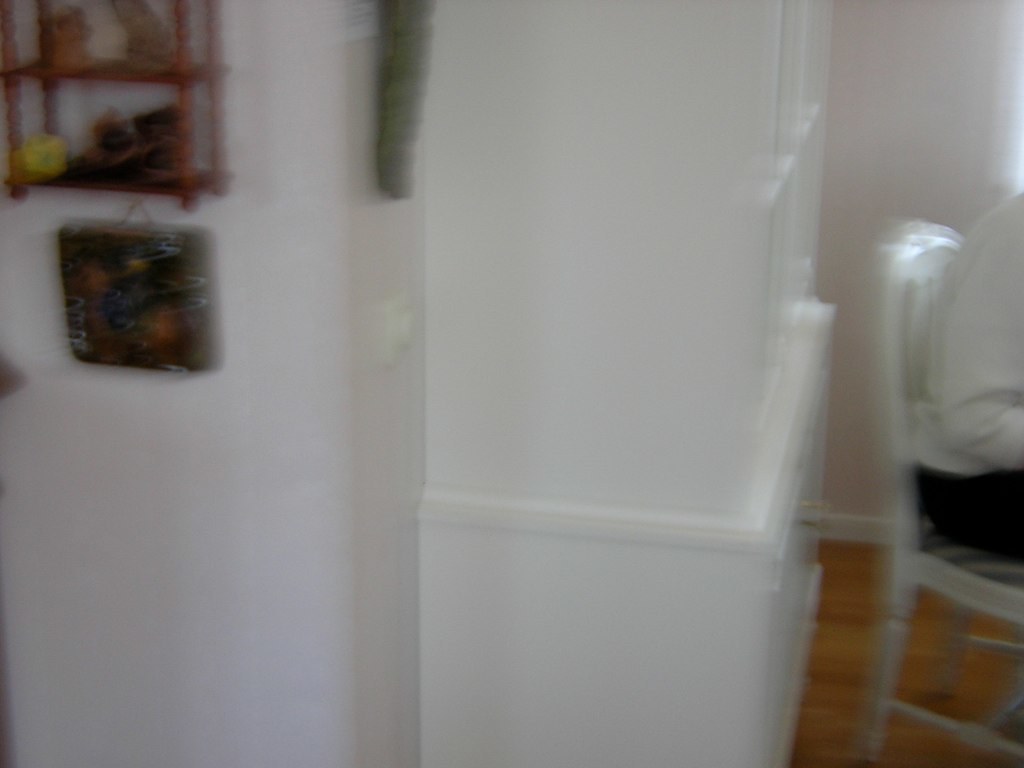This photograph captures a blurry corner of a house, focusing on a segment between what appears to be a kitchen and a dining area. The central focus is a glossy white cabinet, possibly a china cabinet, viewed from the side. To the right of the cabinet, there is a white dining chair with a striped seat, partially occupied by a person in a light gray sweatshirt and black pants, leaning slightly. The walls, covered in a light gray hue, sport a dimmer switch and a small wooden curio shelf in the top left corner, housing several small statues. Below the shelf is a square, dark-colored plaque with lines and dark blue detailing. The flooring is a medium brown hardwood, complementing the soft, neutral tones of the room.